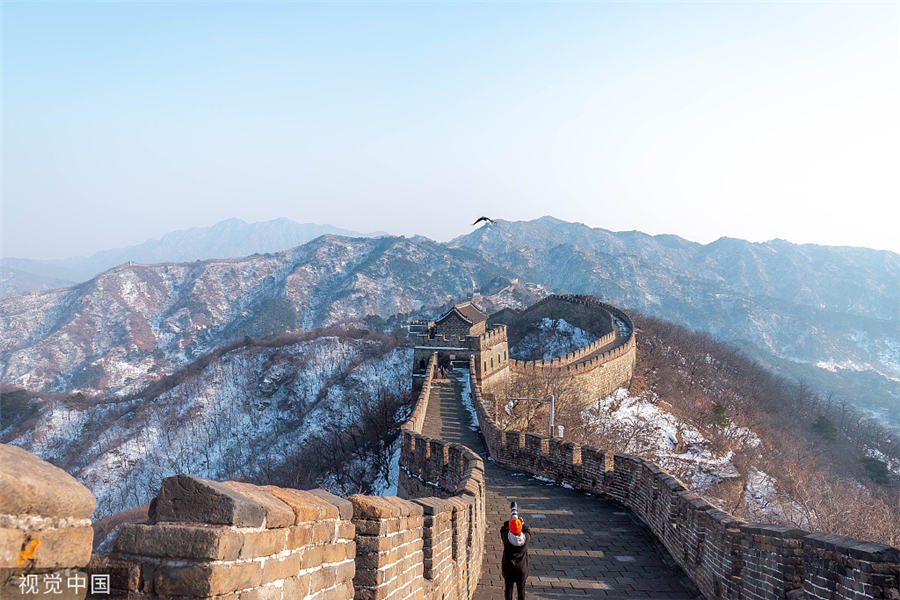In this wide-angle photograph of the Great Wall of China, taken from a high vantage point on the wall's walkway, the viewer's eye is drawn to a person 30 feet below wearing a black jacket and an orange cap. This individual is holding a wide-angle lens, capturing a paraglider soaring over the snow-covered mountains and a segment of the wall itself. The Great Wall meanders towards a guard post halfway into the photo and continues to stretch into the mountainous background, which is dusted with frost and snow. The early morning sun rises over the mountains, casting a warm glow on the blue sky and illuminating parts of the landscape. Detailed bricks of the wall are visible, surrounded by snow and frost, contributing to the wintery ambiance. Additionally, there are four Chinese text symbols in the bottom left corner of the image, adding an authentic touch to the scene.